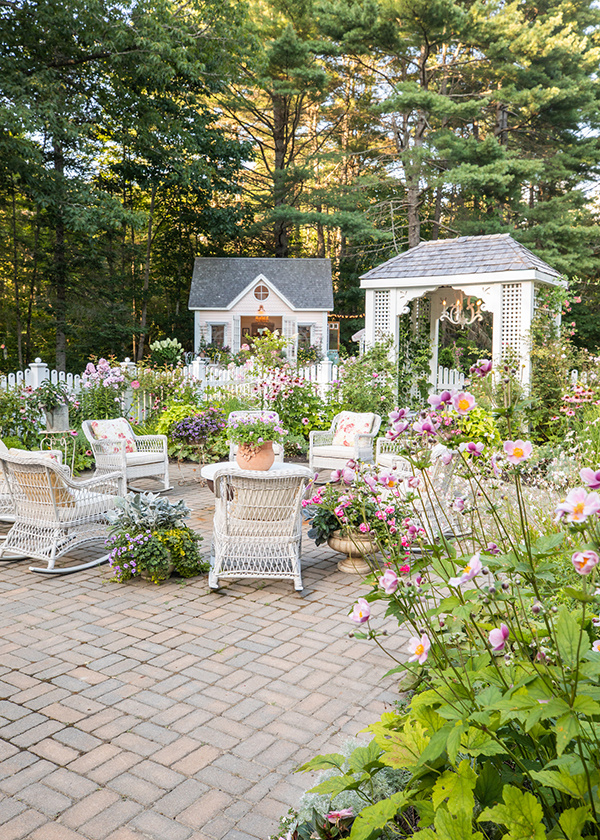The image depicts a picturesque garden setting, ideal for a wedding venue. The scene is centered around a brick patio with a curved edge, surrounded by blooming flowers in purple, pink, and white hues, all set against a lush woodland backdrop. Seven white wicker rocking chairs, each adorned with cushions, are thoughtfully arranged in a circle on the brick surface, interspersed with planters brimming with greenery. In the middle of the arrangement stands a matching white wicker table, also adorned with a planter overflowing with vibrant plants. The garden also features a charming white trellis arch, woven with climbing vines, leading to a quaint white shed with a peaked roof and delicate windows. The entire area is bathed in sunlight, enhancing the serene and inviting ambiance of this enchanting garden.